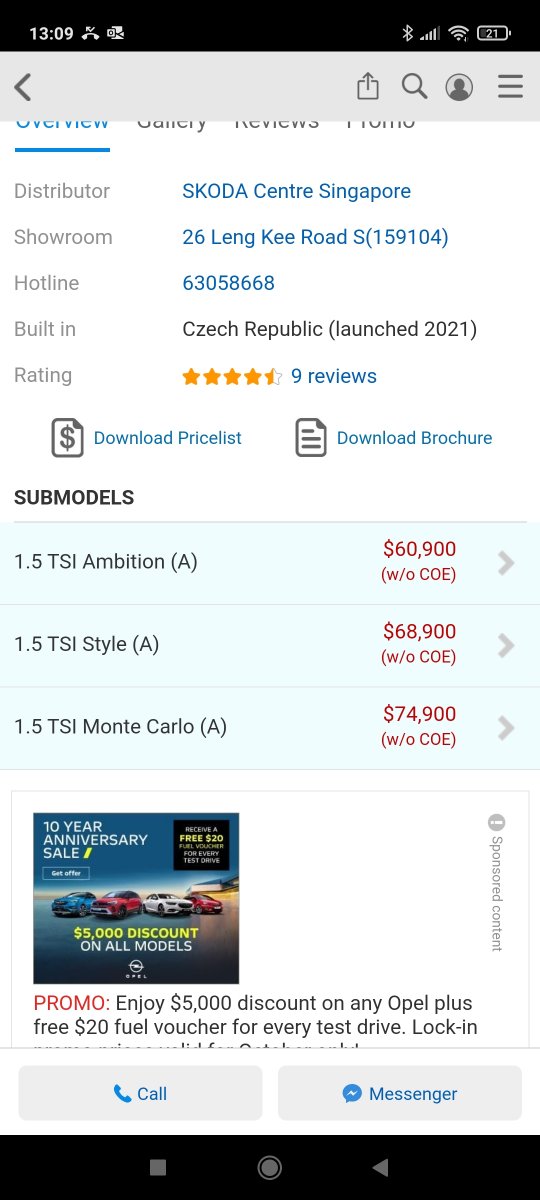The screenshot depicts an Android device displaying a detailed webpage for a Skoda car dealership. 

At the top of the screen, there's a gray header bar containing various navigation buttons: a back button, a share button, a search button, a profile button, and a hamburger menu to reveal additional options. 

The main content of the webpage introduces the dealership as the "Skoda Center, Singapore" located at "26 Leng Kee Road, S" with a hotline number "63058668". The Skoda vehicles are depicted as being "built in the Czech Republic" and launched in "2021".

The webpage also lists several vehicle models, including the "1.5 TSI Ambition", "1.5 TSI Monte Carlo", and their respective prices: "$60,000", "$68,000", and "$74,900". 

Scrolling down, there's an advertisement for a "10-year anniversary sale" with a "$5,000 discount on all models". The ad features images of four cars displayed horizontally. Additionally, it promotes an offer of a "$5,000 discount on any Opel" plus a "free $20 fuel voucher for every test drive". Some text in the advertisement is cut off and not visible.

Below the ad, there are two buttons: one labeled "Call" which presumably initiates a phone call to the dealership, and another labeled "Messenger" which likely opens a Facebook messaging chat with the dealership.